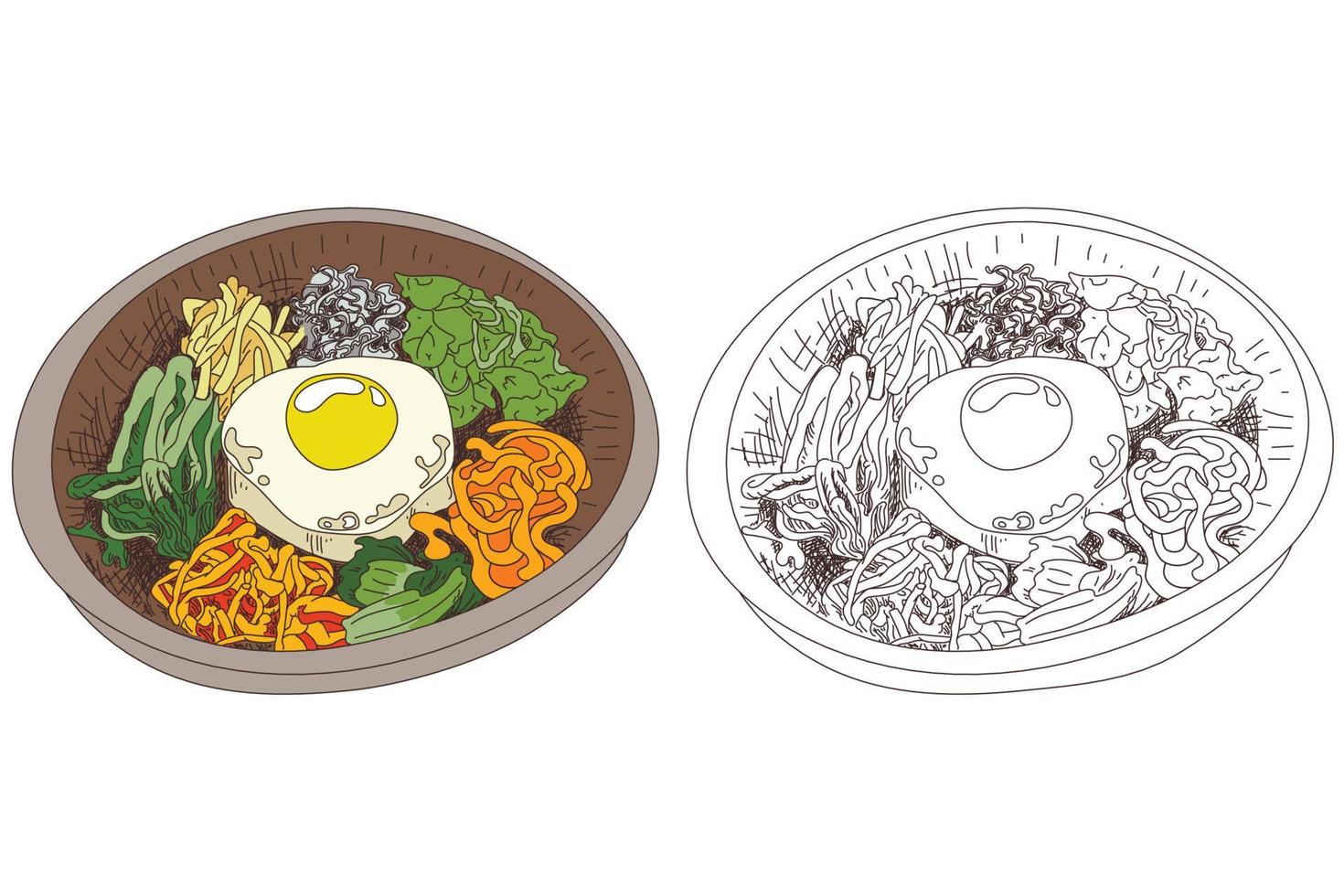The image depicts two side-by-side drawings of the same dish, set in a brown bowl. The left drawing is in full color, while the right is a black-and-white line art version with a slight brownish tint. At the center of both drawings is an egg with a prominent yellow yolk surrounded by white. The egg is placed in the middle of an omelet. Surrounding the egg, the dish contains various vegetables and other food items: several green leaves, possibly celery or lettuce; pieces of orange carrots; items with both light and dark orange hues; and deep reddish-colored foods. The colored drawing distinctly shows the vibrant hues of these ingredients, while the black-and-white version uses various shades of gray and brownish black to illustrate the same details.